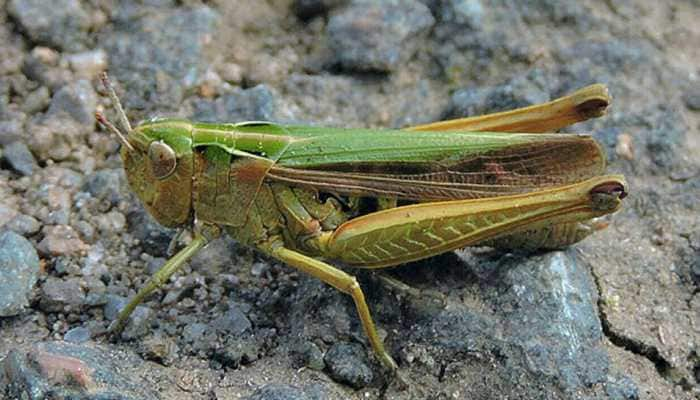The image features a close-up of a grasshopper centrally positioned both vertically and horizontally. This vivid creature, primarily displayed in various shades of green—from dark to light—captures the eye. Its folded wings exhibit a brownish hue, while its body transitions from green on its upper parts to a golden and orange-ish-yellow tone on its lower segments. The grasshopper's delicate antennae and legs, with golden hues, are clearly visible, especially the front legs which occupy the bottom left portion of the image. The terrain, upon which the grasshopper rests, appears to be a combination of dry, cracked dirt with scattered pebbles and rocks, colored in browns, grays, slight blues, and even a tinge of reddish-brown. The background further emphasizes the rough, arid nature of the landscape, devoid of any other objects or creatures. This beautifully composed image meticulously captures the intricate details of the grasshopper in its natural habitat.